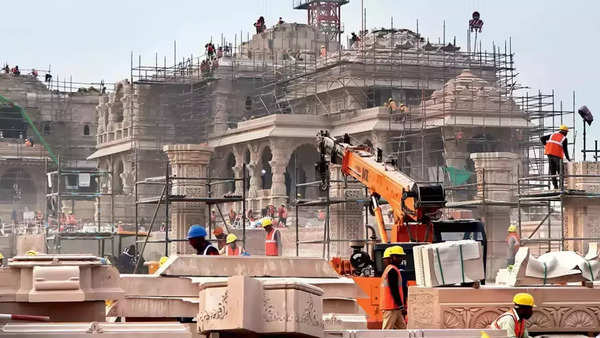The image captures an extensive and bustling excavation site, likely an archaeological dig or restoration project of an ancient stone structure. The central structure showcases intricate architecture, including multiple stone archways and elaborate pillars that rise through at least three levels. Surrounding this focal point are layers of metal scaffolding, indicating ongoing work and preservation efforts. 

In the foreground, massive carved stone blocks feature detailed carvings—depicting suns, eagles, and looping patterns—possibly hinting at the cultural or historical significance of the site. Nearby, an orange crane with a retractable arm is positioned near these carved blocks, suggesting active construction work.

To the left of the main structure, another large edifice is enveloped in scaffolding and appears to be part of the same excavation project. The site teems with construction workers, identifiable by their orange safety vests and yellow or blue hard hats, emphasizing the collaborative effort and scale of the operation. The workers’ dark skin and the potential architectural style hint that the site might be located in a Middle Eastern or Asian region. The photo, taken with a light sky in the background, captures a bright midday scene filled with industrious activity.